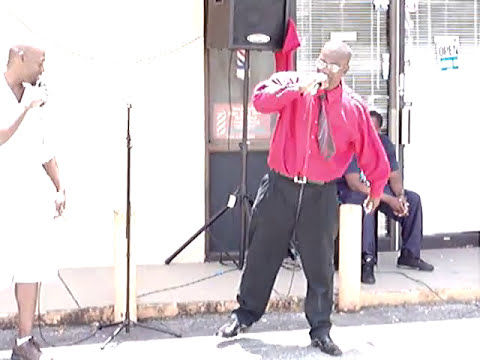In this vibrant street performance scene, two African-American men captivate the public on a bustling sidewalk. On the left, a man in a white shirt and white shorts, paired with brown shoes, looks intently to his left, where his fellow performer stands. This performer, positioned to the right side of the image, is attired in a striking red long-sleeve shirt, a black and red tie, black pants, and black shoes. He holds a microphone in his right hand, wears glasses, and is bald. Behind him stands a large black speaker mounted on a tripod. To complete the scene, a third man dressed in a navy blue outfit sits clasping his hands in front of a door marked with an 'Open' sign, framed by windows with blinds. The setting appears to be outdoors, contributing to the lively street ambiance.